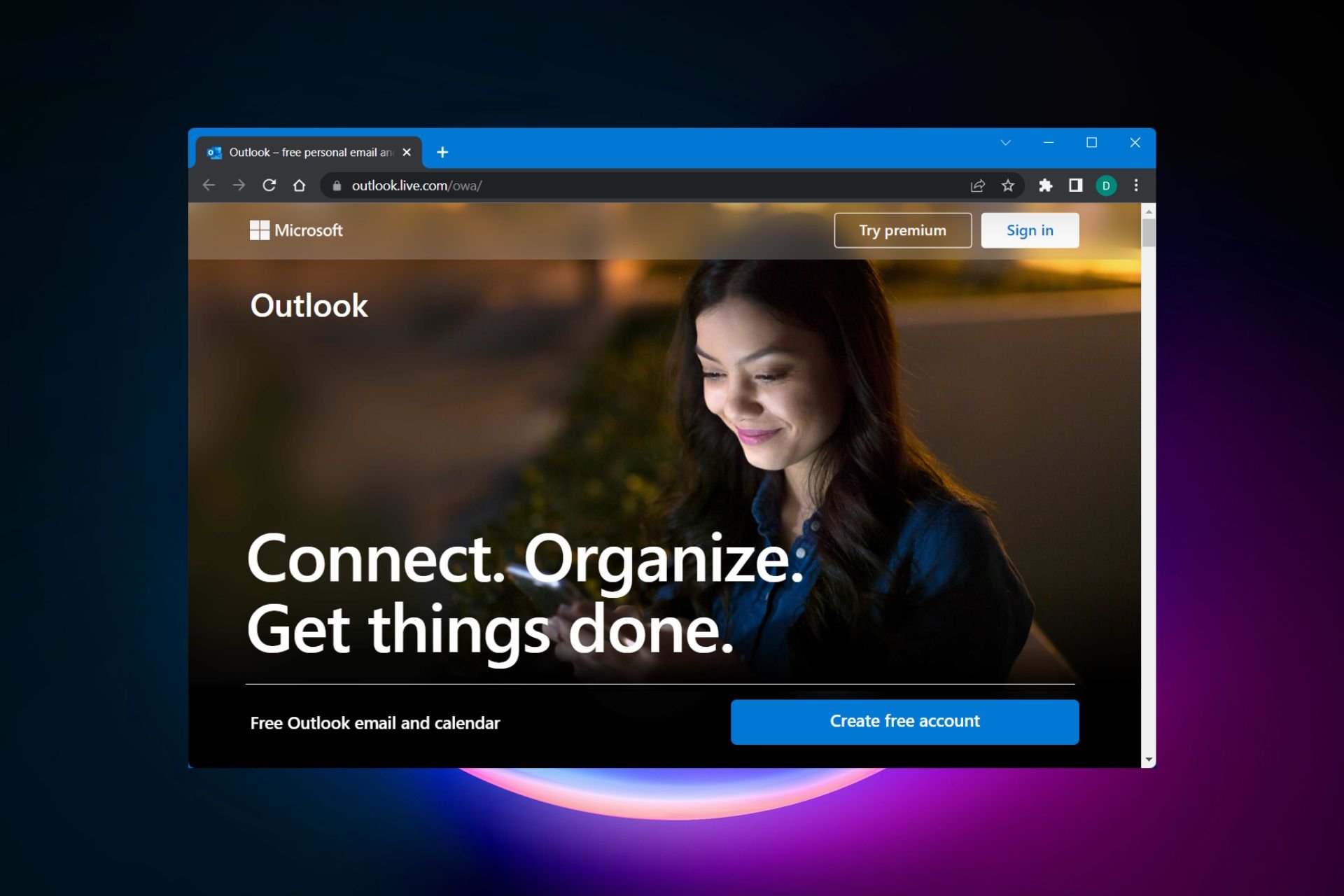The image showcases a screenshot of a Microsoft webpage, specifically the Outlook login page. The overall design features a dark black border at the top, transitioning to a very dark blue on the left side and a purple hue on the right side of the background. The screenshot sits centrally within these borders, displaying the full browser window.

At the top of the browser window, a blue bar clearly indicates the web address, which is "outlook.live.com." The top left corner of the webpage displays the word "Microsoft" alongside the Windows logo, both in white. On the right side of the header, there are three links: "Sign up," "Sign in," both in white, and "Try Premium," which is outlined.

Dominating the page, there is a large photograph of a woman, depicting her head and upper shoulders. She appears to be in her late twenties or early thirties, has long brown hair, and is wearing a dark blue shirt. She is looking down at her smartphone. The headline positioned to the left of the image reads "Connect. Organize. Get things done," in white font. In the lower right corner, there is a blue rectangle with the text "Create free account" in white.